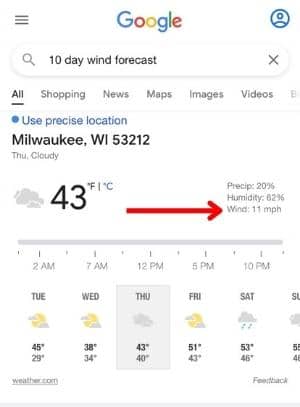**Detailed Caption:**

This is a screenshot captured from a smartphone displaying a weather forecast. At the top, it shows the Google search bar with various options such as "10-day wind forecast," "Off," "Shopping," "News," "Maps," "Images," and "Videos." An option to "Use precise location" is also visible. The location specified is Milwaukee, Wisconsin, ZIP code 53212.

The weather information is centered on a forecast for Thursday, indicating it will be cloudy with a temperature of 43 degrees Fahrenheit. A prominent red arrow points to the wind speed, which is 11 miles per hour. Additional weather details include 62% humidity and a 20% chance of precipitation.

Beneath this, there's a five-day forecast:
- Tuesday: 45 degrees Fahrenheit
- Wednesday: Partly Sunny, 38 degrees Fahrenheit
- Thursday: Cloudy, 43 degrees Fahrenheit
- Friday: Partly Cloudy, 51 degrees Fahrenheit
- Saturday: Rain, 53 degrees Fahrenheit

The data source is weather.com, and a "Feedback" option is also displayed.